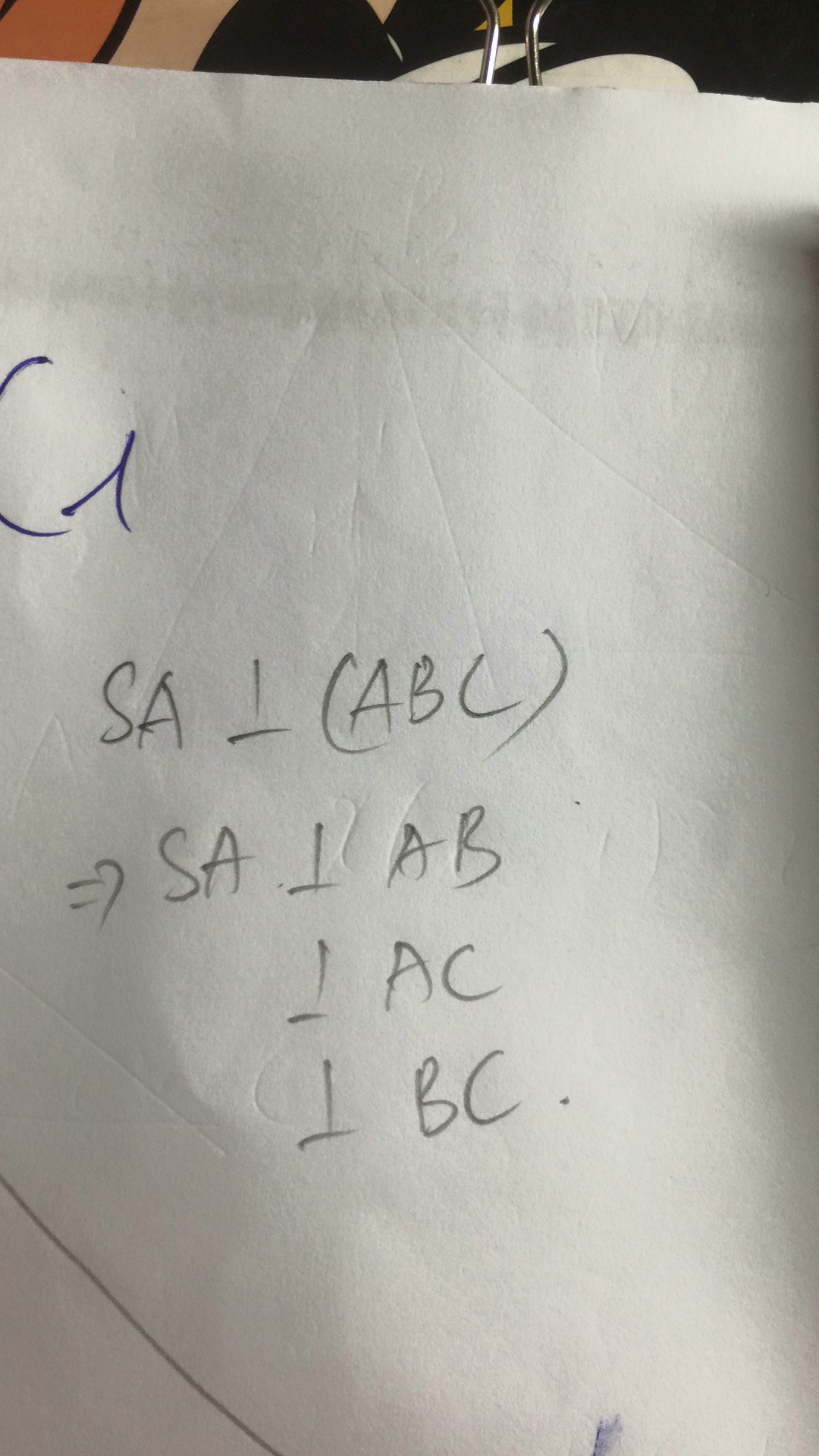In this portrait-oriented close-up photo, various scribbles and mathematical or programming-related notes are visible. At the very top left, there's a hastily written letter "G". Beneath this, the paper shows indents suggesting it was underneath another sheet when someone was writing. 

Further down the first row, the notation starts with "SA" followed by an upside-down "T" and the text "(ABC)" inside parentheses. Below this, the sequence continues with "= 7 SA" along with the upside-down "T" symbol and "AB". The pattern maintains as the next line features an upside-down "T" with "AC". This is followed by yet another line with the upside-down "T" accompanied by "BC...".

In the bottom left corner, a line stretches horizontally across the paper, seemingly insignificant. Lastly, in the bottom right corner, there's a notable dark blue smudge. At the very top of the photo, a minor sliver of the background is visible, though it is too faint to discern any details.